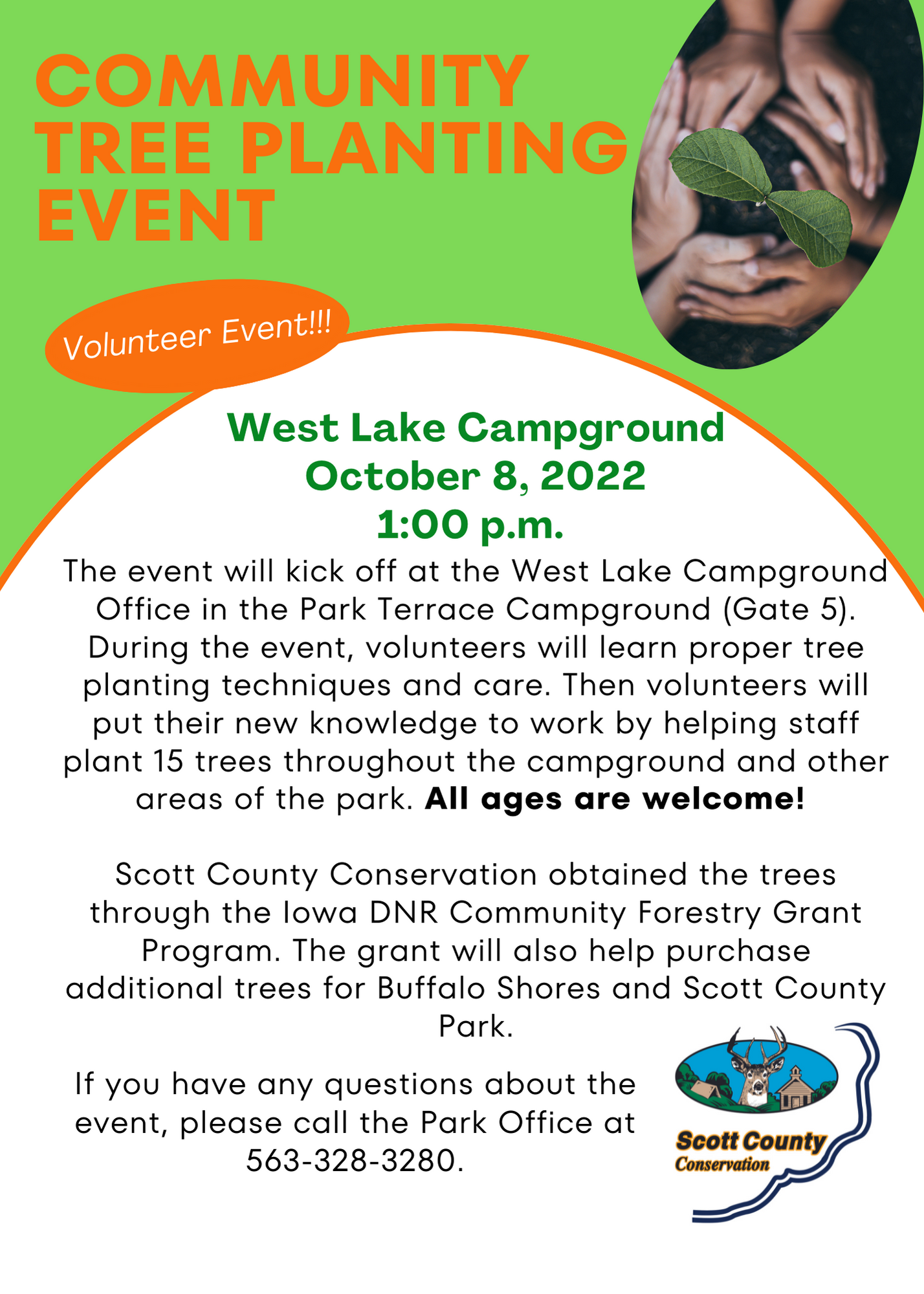This is a brightly colored flyer for a Community Tree Planting Event on October 8th, 2022, at 1 p.m. at Westlake Campground. The top of the flyer features a light green background with the event title in bold orange text. An oval in the top right corner depicts several pairs of hands cupping a small green plant on a black background. Below, green text indicates the event specifics: "Westlake Campground, October 8th, 2022, 1 p.m." 

Detailing the event, black text explains that it will kick off at the Westlake Campground office in the Park Terrace Campground, Gate 5. Participants will learn proper tree planting techniques and care, then apply their new knowledge to plant 15 trees across the campground and other park areas. The message boldly notes, "All ages are welcome!"

Sponsored by Scott County Conservation, the event's trees were obtained through the Iowa DNR Community Forestry Grant Program, which will also fund additional trees for Buffalo Shores and Scott County Park. The bottom right corner of the flyer features the Scott County Conservation logo, depicting a deer among buildings, trees, and a blue sky. For questions, the park office contact number is 563-328-3280.